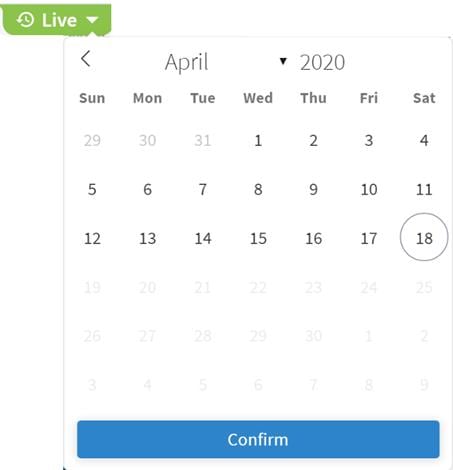The image captures a partial view of a website displaying a calendar interface. The top section shows the word "Live" in green text, accompanied by a drop-down arrow button. Next to it, there's an icon resembling a clock with a circled arrow around it, also labeled "Live." Below this header, an arrow pointing left, positioned within a box, likely functions to navigate to the previous month, as the highlighted month displayed is April. On the right side, an arrow pointing downward is located next to the year "2020," likely used for changing the year.

The main body of the calendar includes the days of the week—Sunday, Monday, Tuesday, Wednesday, Thursday, Friday, and Saturday—listed in a smaller, bolded black font. The calendar grid begins with the final three days of the previous month, labeled 29, 30, and 31, which appear under Sunday, Monday, and Tuesday respectively and are lightly faded in gray. The dates continue sequentially in bold black font up to the current date of the 18th, while the remaining dates for the rest of the month are faded to indicate they are not selectable. At the very bottom of the calendar is a confirm button.